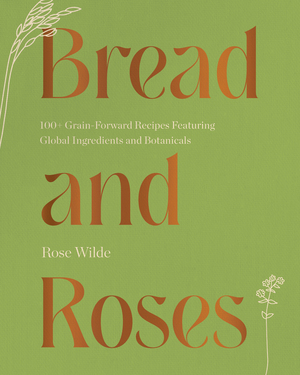The cover of the book "Bread and Roses" features a vivid lime green background with a striking and decorative title in large, easy-to-read red lettering. The words "Bread" and "Roses" are prominently displayed, separated by the word "and" in a similarly eye-catching style. Below the title, the subtitle, "100+ Grain-forward Recipes Featuring Global Ingredients and Botanicals," is elegantly printed in a lighter font. The author's name, "Rose Wild," is also visibly noted in white. 

The artistic elements on the cover include intricate white designs of grain stalks with tiny leaves positioned at the top left and bottom right corners, adding a natural and botanical touch to the overall design. The combination of the vibrant background, detailed fonts, and botanical illustrations creates an inviting and visually appealing cover, making it stand out as an intriguing read for those interested in cooking with global ingredients and grains.